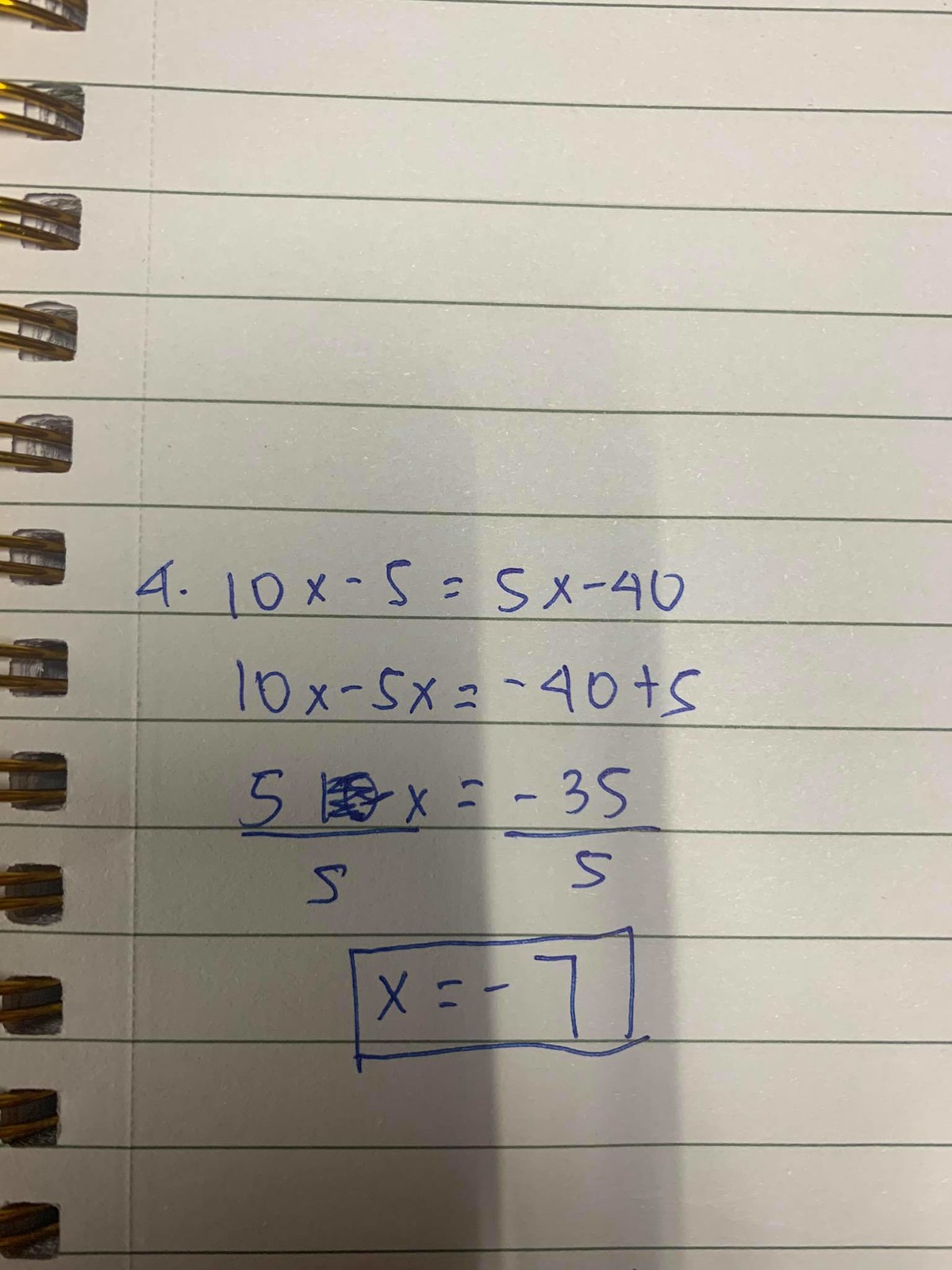This zoomed-in image captures a piece of white notebook paper with light gray lines and holes along the left-hand side, suggesting it is part of a metal-bound notebook that's been opened. The medium blue ink equations span approximately four lines, culminating in a boxed answer. The equation prominently reads "10x - 5 = 5x - 40" or it might be "90". The subsequent line simplifies to "10x - 5x = -40" or possibly "-90" plus 5, resulting in "5x = -35". This is further divided to reveal the final answer "x = -7", neatly boxed at the bottom. A long, dark rectangular shadow darkens the bottom left of the page, gradually fading into a lighter shade and casting over part of the equation and the final answer.